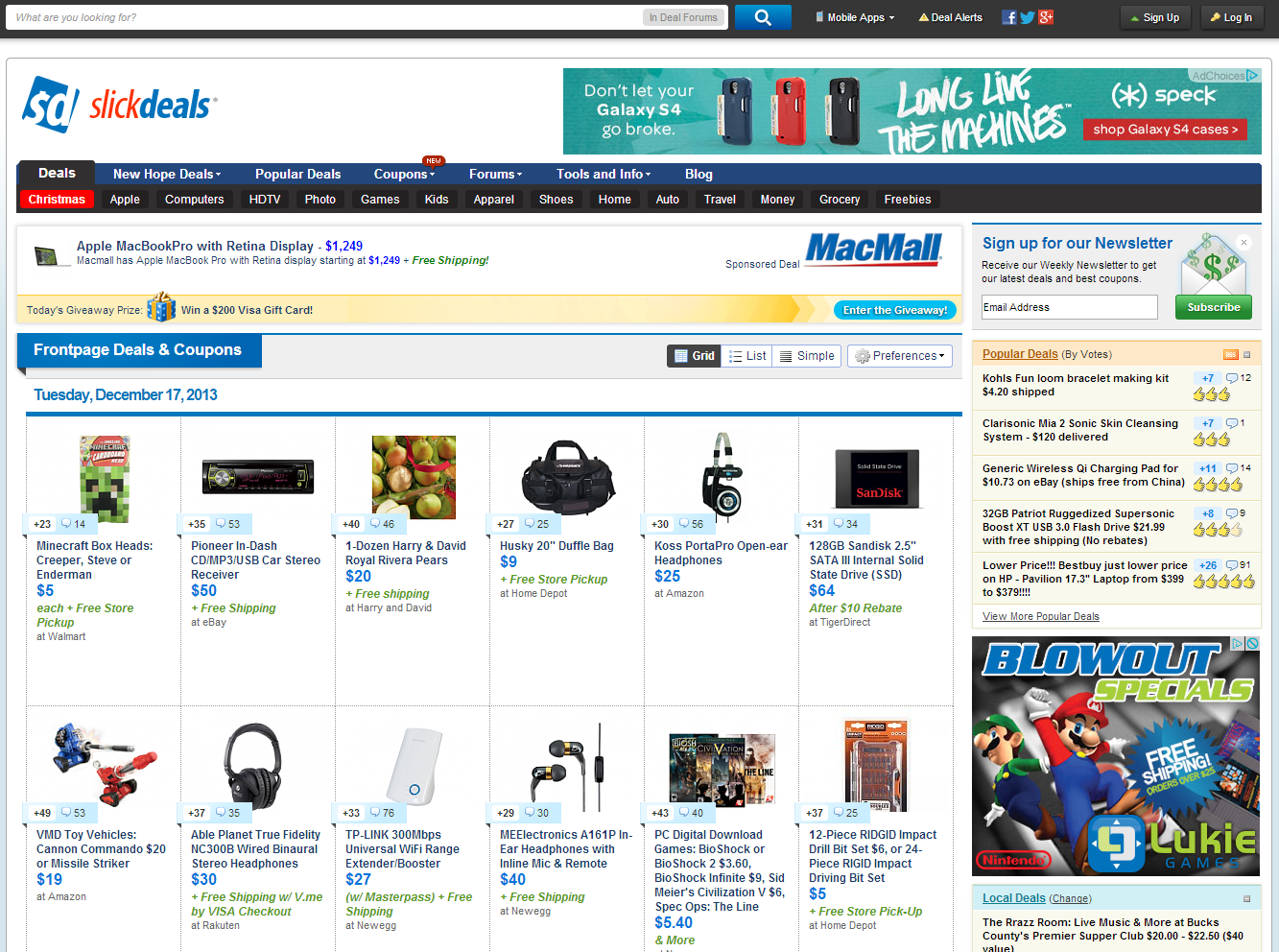This image is a screenshot of the website "Slick Deals" captured on Tuesday, December 17, 2013. In the upper left corner of the screen, there is a combined search and address bar with the prompt "What are you looking for?" in light gray text. To the right of the search bar, there are quick links labeled "Mobile Apps," "Deal Alerts," "Facebook," "Google," "Twitter," and "Login."

At the top left section of the page, the website's name "Slick Deals" is prominently displayed. Adjacent to this, there is an advertisement featuring three cell phone cases intended for the Galaxy S4, with the tagline "Don't let your Galaxy S4 go broke. Long live the machines. Spec. Shop Galaxy S4 cases."

Below the advertisement, the main content highlights various "Front Page Deals and Coupons" for the day. The deals include:

- **Minecraft Box Heads (Creeper, Steve, or Enderman):** Priced at $5 each with free in-store pickup at Walmart.
- **Pioneer In-Dash MP3/USB Car Stereo Receiver:** Available for $50 with free shipping on eBay.
- **One Dozen Harry and David Royal Riviera Pears:** Priced at $20 with free shipping from Harry and David.

This detailed screenshot captures the essence of Slick Deals’ interface, along with a variety of attractive offers available on that particular day.